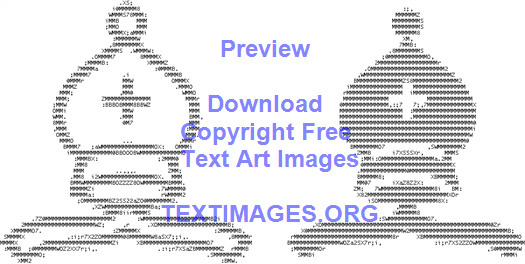The image presented is a digitally synthesized artwork featuring two intricate symbols reminiscent of crowns, created using word art or lines composed of small alphanumeric characters. The two symbols, identical in size, occupy the left and right sides of the image against a white backdrop. Each crown-like symbol boasts a teardrop-shaped head and a small square base. From the base, delicate swirls extend outward in both directions, resembling tentacles.

The symbol on the right is a filled design, where the lines of text or numbers intricately fill the interior, save for a white cross at its center. The symbol on the left, in contrast, is an outlined version of the crown, with the center cross shaped by the aggregation of individual letters or numbers, and the rest of the crown remaining white.

Overlaying the image, in a transparent blue text, is the phrase: "Preview, download copyright-free text art images, textimages.org."